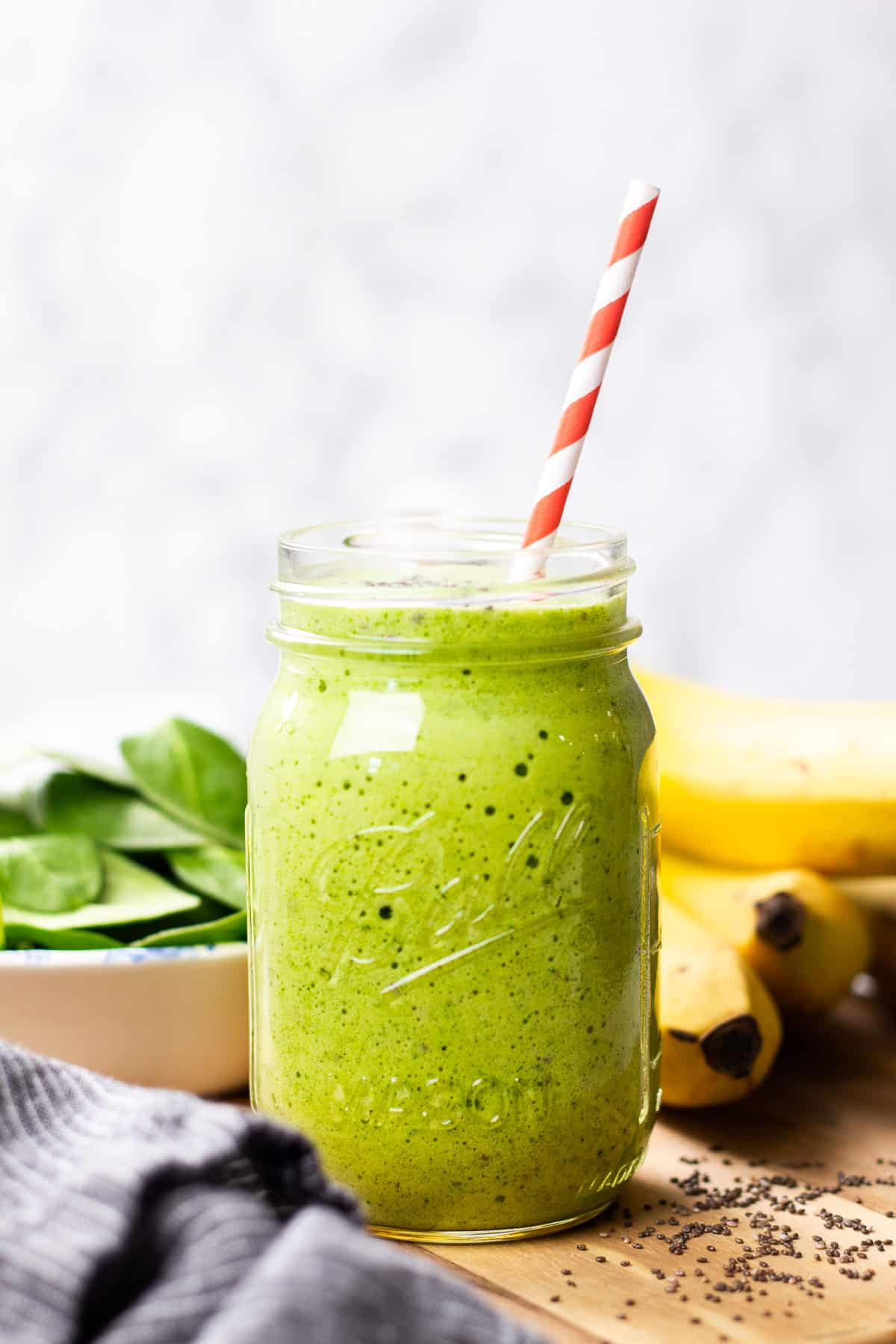This photograph showcases a vibrant and aerated green smoothie, presented in a classic mason jar. Adorning the smoothie is a strikingly red and white diagonally striped paper straw, reminiscent of a candy cane, which stands upright, indicating the drink's thick consistency. Surrounding the jar is an artfully arranged scene: to the foreground, seeds presumed to be acai or poppy seeds are scattered on a wooden cutting board beside a navy blue kitchen towel. In the background, ripe bananas lay behind the jar, adding a fresh touch, and a white bowl filled with spinach leaves sits to the left, suggesting these ingredients are part of the smoothie’s composition. The image is set against a gray and white abstract backdrop, lending a stylized, staged quality to the presentation.